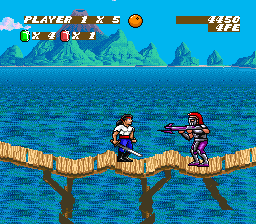This image captures a highly pixelated, retro-style video game scene set on a rickety wooden bridge spanning a large, dark blue body of water. In the distance, tall, pointy-tipped mountains rise against a blue sky dotted with a white cloud. The central focus is on two characters standing on the bridge. To the right, a man with blue jeans, a white shirt, black calf-high boots, and a red belt stands ready with a silver sword in hand. He has blue eyes and wears a red headband. Opposite him, a futuristic figure, potentially a woman, brandishes a silver and purple gun. This character sports a red mohawk and silver and purple armor. At the top left of the screen, "Player 1 x 5" is displayed in white text on a brown background. Next to it, icons show a green gem "x 4" and a red crystal "x 1." The top right corner features a number sequence, "44504 FE." The scene vividly evokes the aesthetic of video games from the 1990s to early 2000s.